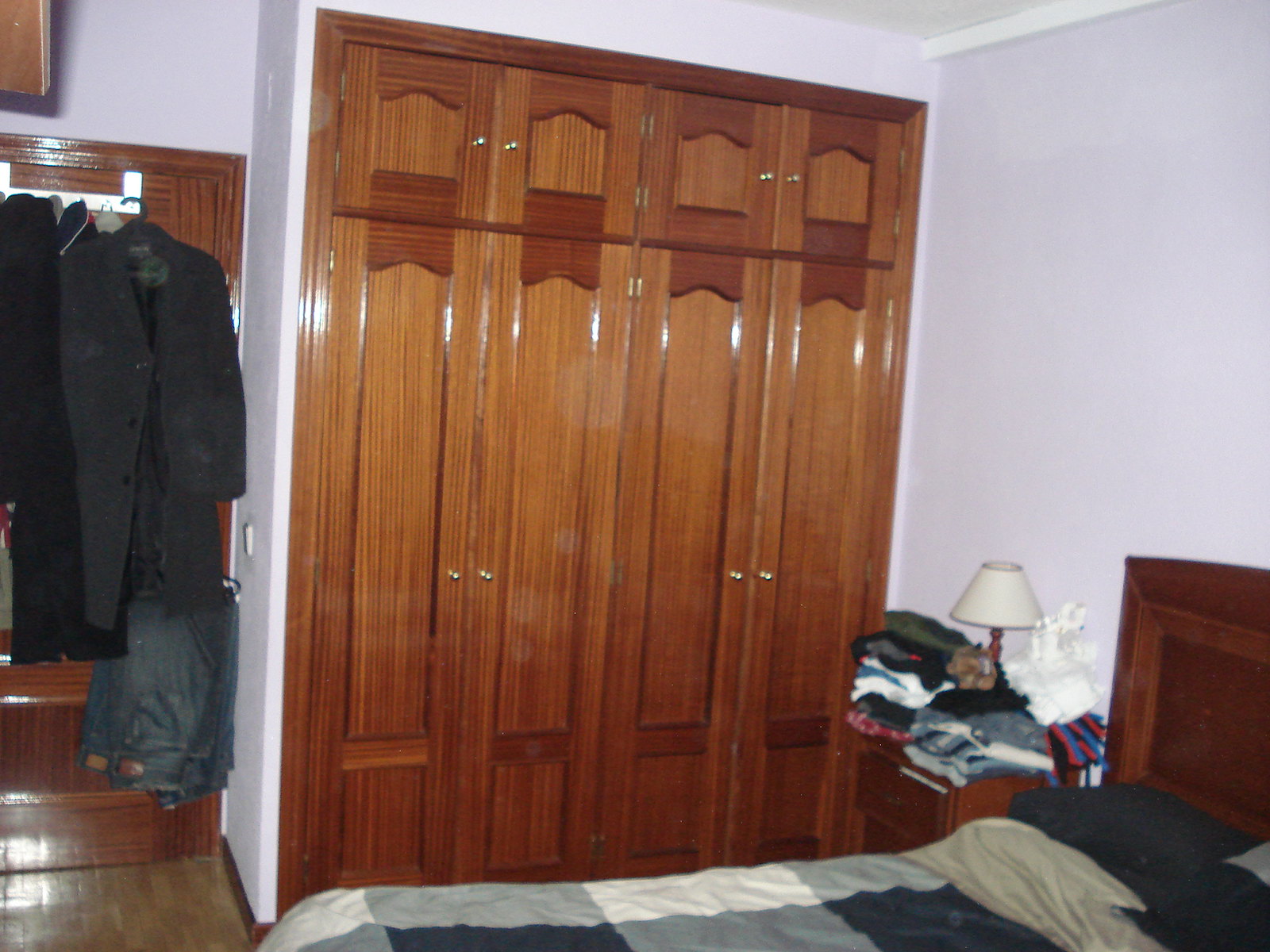This color photograph of a bedroom showcases a space with violet walls prominently featuring beautifully refinished closet doors. The closet consists of two sections, each with four doors, making up two comprehensive sections of tall, narrow, and shiny wooden doors. The wood is stained a rich brown with some sections incorporating a deeper chocolate brown hue at the top, and all doors are adorned with small, reflective brass knobs. The wooden frame around the closet matches the doors' color.

Adjacent to the closet, on the left, a white metal rack with hooks holds an assortment of black clothing, including suit jackets and jeans. Behind this, there is an armoire that mirrors the closet's brown tones, melding light and dark browns.

The bed situated in the foreground has a headboard of chocolate brown wood and is dressed in a white, gray, and black checkered comforter, complemented by a pillow in a black case. To the left of the bed is a small wooden nightstand with drawers that share the same chocolate and lighter brown color scheme as the other wooden furniture in the room. This nightstand is overwhelmed with folded clothes and supports a small wooden lamp with a curved white lampshade. This detailed setup creates a cohesive and rich visual experience in the entire bedroom.